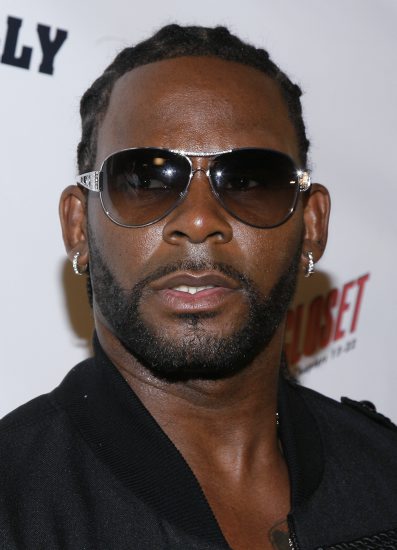This is a professional photograph of R. Kelly, taken at a celebrity event in front of a white backdrop with red and black writing, including the partially visible text "LY," "closet," and some unreadable lines beneath. R. Kelly, known for his controversial rap opera "Trapped in the Closet" among other infamies, is facing the camera but looking slightly to his right, avoiding direct eye contact with the photographer. He has a serious expression with a slightly open mouth revealing the edges of his bottom teeth. His hair is styled in signature braids, and he sports tinted sunglasses, likely encrusted with diamonds, along with diamond-studded earrings shaped like the letter C in both ears. His well-groomed goatee complements his rich cocoa skin, which appears shiny as if he's a bit sweaty. He is dressed in a black jacket left open to reveal a partial chest tattoo, indicating he isn't wearing a shirt underneath. The image captures his well-known public persona with meticulous detail.